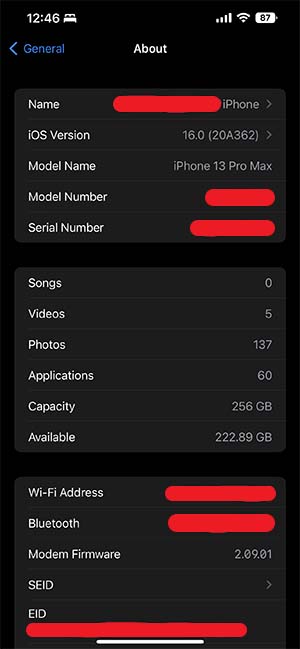A detailed screenshot of an iPhone 13 Pro Max's "About" settings page. It shows the device connected to Wi-Fi with a full signal and a battery level of 87%. The time displayed is 12:46. The owner's name is partially redacted, revealing only "iPhone" at the end. The software version is iOS 16. Specific details like the model and serial numbers are highlighted and thus obscured. The device's storage capacity is 256 GB, with 222.82 GB available. The user has no songs, five videos, 137 photos, and 60 apps installed. Fields for the Wi-Fi address and Bluetooth are grayed out. Modem firmware is listed as a series of numbers. The SEID field has a clickable arrow, while the EID is marked with a red line, indicating its presence.